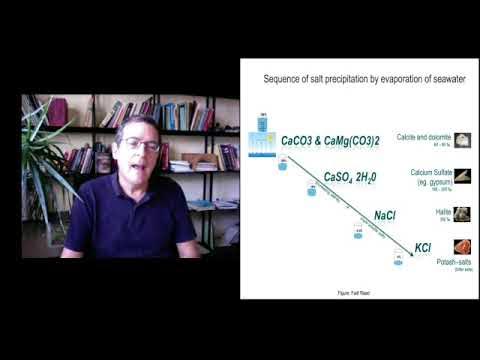In the image against a solid black background, on the left-hand side, there is a photograph of an academic-looking man who appears to be mid-sentence, hinting at an interview or a presentation. He is seated, wearing glasses and a blue polo shirt. His dark hair and the slightly untidy office environment add to the casual and informal feel of the setting. Next to him, a green plant with pointy leaves, likely an aloe plant, adds a touch of nature. Behind him, a tall bookshelf crammed with books tipping over to the sides showcases a workspace filled with research materials. On the right-hand side of the image is a detailed diagram, titled "Sequence of Salt Precipitation by Evaporation of Seawater." This diagram includes a descending line marked with various chemical formulas like CaCO3 (calcium carbonate), CaMg(CO3)2 (dolomite), CaSO4·2H2O (gypsum), NaCl (sodium chloride), and KCl (potassium chloride). The diagram features text in varying shades of blue, and at its bottom, there are three small words that are barely readable. This setup suggests that the man is discussing his research findings on salt precipitation during the evaporation process of seawater, perhaps in an educational video or a recorded lecture.